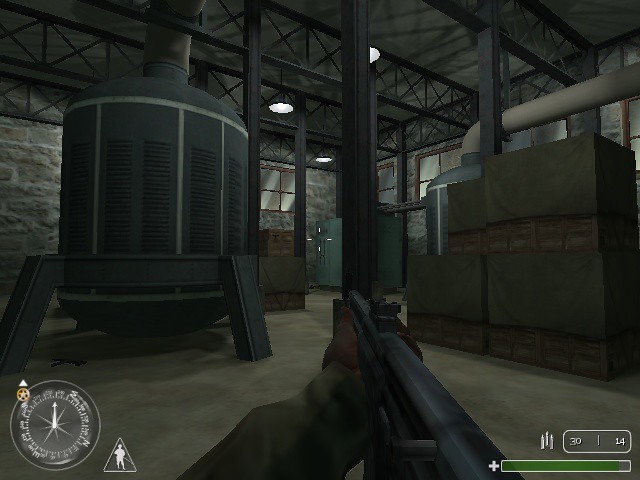This detailed screenshot from a first-person shooter video game captures a dark, industrial factory or basement-like environment. The scene is dominated by exposed steel posts, steel girders, and grayish stone walls, contributing to the dim atmosphere illuminated by two white hanging lights that provide minimal brightness. Central to the image is a large black, circular boiler, with additional industrial equipment, possibly air conditioning units or water heaters, visible on both the left and right sides. The right side also features a pipe extending from the machinery. Several brown boxes covered with green tarps are scattered around, adding to the cluttered feel of the room. The player's perspective shows an arm with a green sleeve and a brown-gloved hand holding a long black machine gun, which appears to have a scope. The user interface elements visible include a compass in the bottom left corner, showing the player is facing southwest, a triangle symbol representing a soldier, an ammunition indicator reading "30-14," a white cross, and a nearly full green health bar in the bottom right corner.